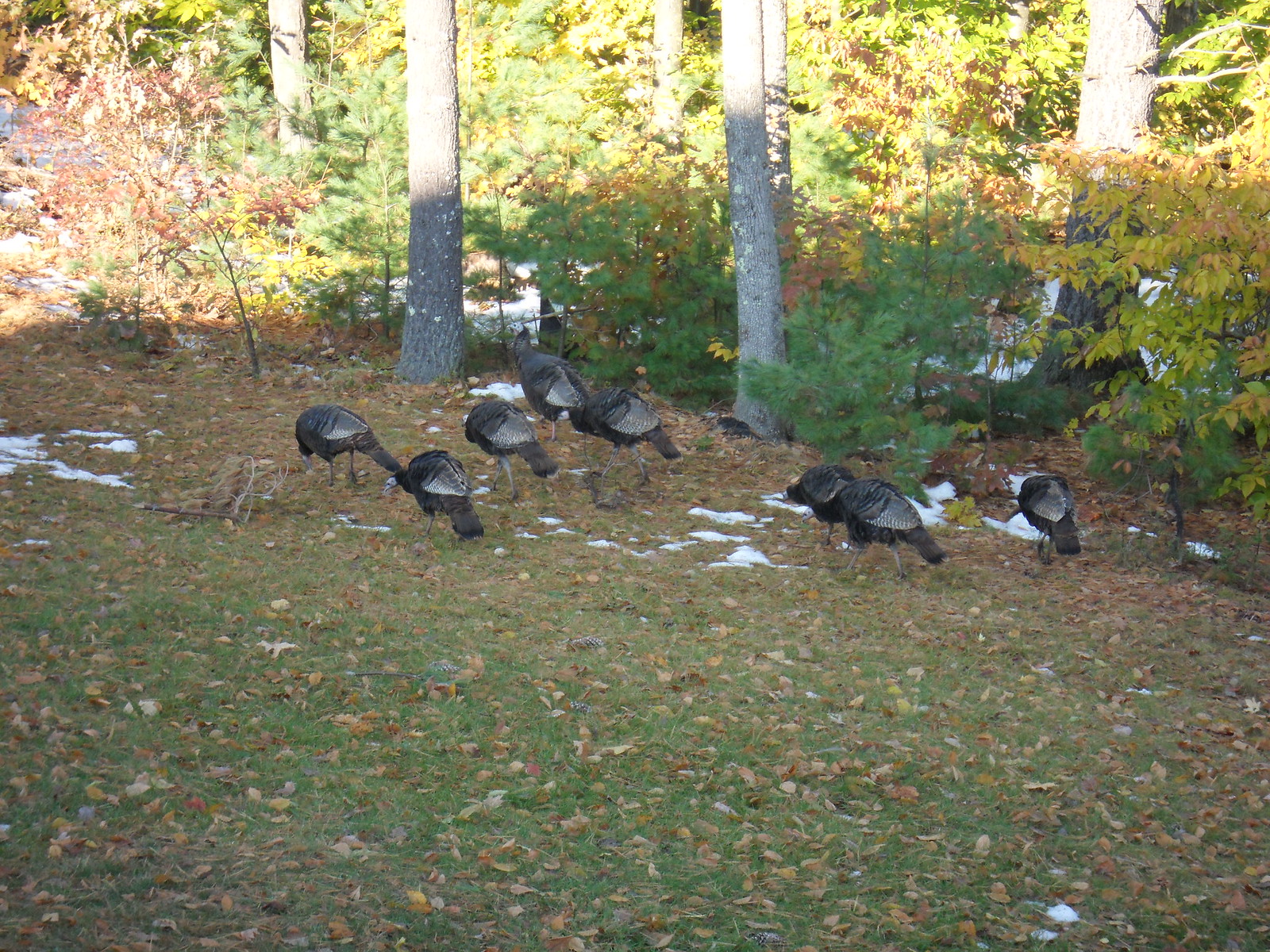This image captures a vibrant autumn scene in a wooded area, showcasing an array of colorful fallen leaves in shades of orange, brown, bright red, and yellow. Scattered amidst the leafy ground are small patches of melted snow. The focal point of the image is a flock of eight wild turkeys, identifiable by their black and silvery-gray striped plumage, and their long, spindle-like legs. Most of the turkeys have their heads down, foraging for food in the grass. The background is filled with a variety of trees and bushes, with some displaying autumn hues of yellow and orange. Shadows cast across the bottom of the image give way to light streaming through the upper parts, highlighting the textured landscape. In the distance, a road is faintly visible beyond the dense foliage.